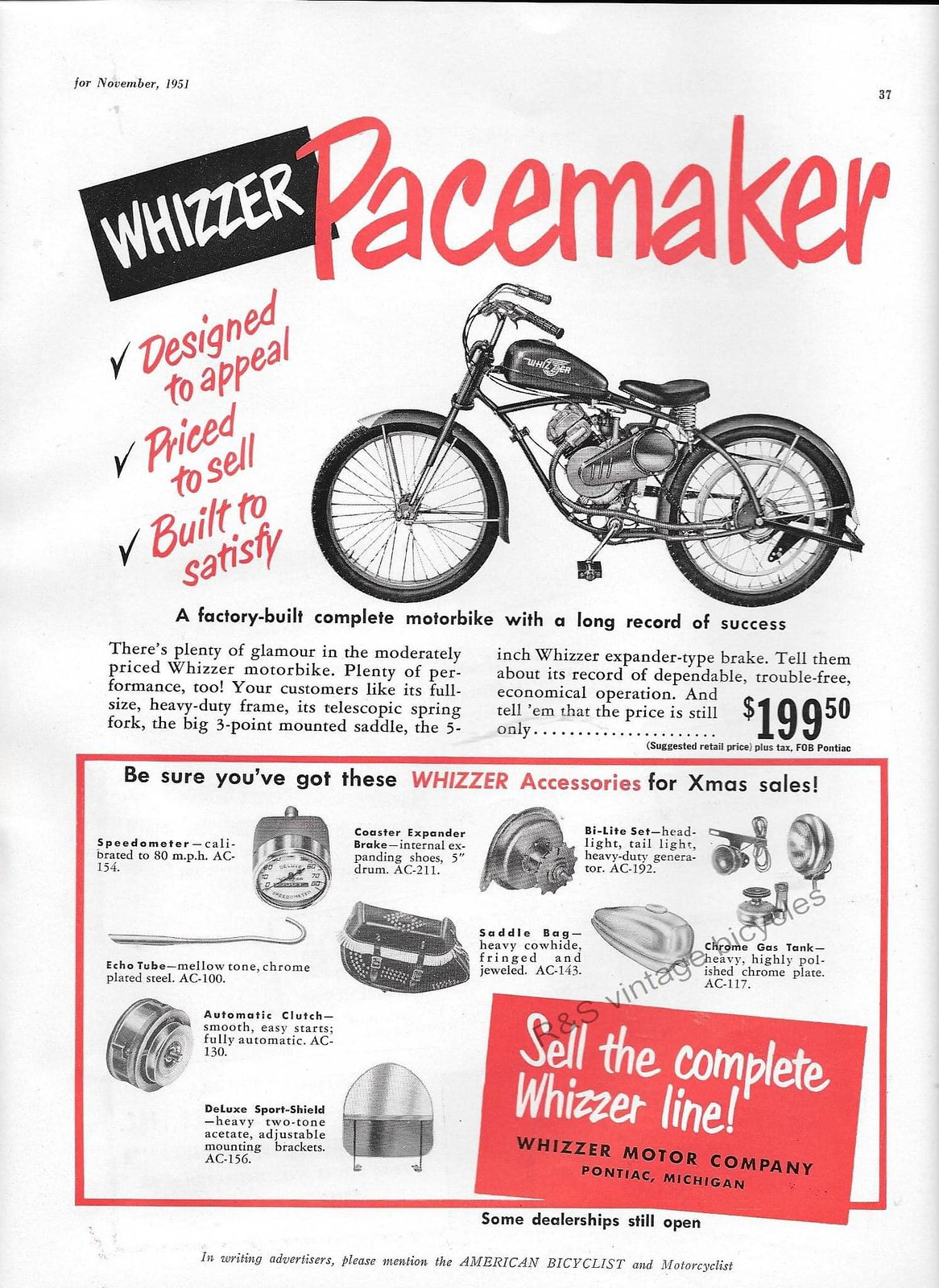This full-page magazine advertisement for the Whizzer Pacemaker, possibly from November 1951 or 1962, emphasizes the slogan "Designed to Appeal, Priced to Sell, Built to Satisfy" alongside a classic motorbike image. At the top of the ad, "Whizzer" is prominently featured in white italic font on a black background, with "Pacemaker" in red, handwriting-style font. A detailed description highlights the factory-built, complete motorbike with a long record of success, priced at $199.50. The ad includes check marks next to the key selling points and a section showcasing additional Whizzer accessories such as a saddlebag, speedometer, echo tube, automatic clutch, and deluxe sport shield, marketed for Christmas sales. The bottom third features a red-bordered bar encouraging viewers to "Sell the complete Whizzer line," with a red diagonal block promoting the Whizzer Motor Company, located in Pontiac, Michigan.